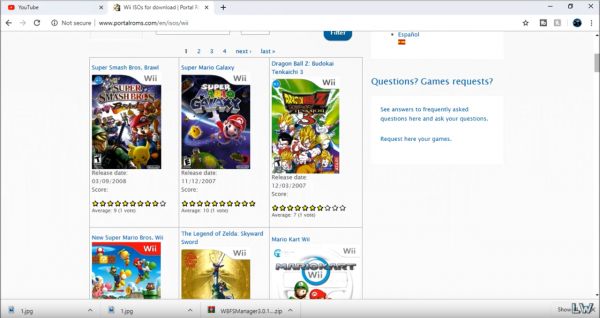On the screen display, a browser tab labeled "YouTube" is visible at the top. The active tab is titled "Y-ISOS for Download Portal." The main section of the screen is divided into a few areas. On the right side, there is a blank space followed by headers labeled "Questions," "Games," and "Requests." Under "Questions," there is text that reads "See answers to frequently asked questions here and ask your questions." Under "Requests," it says "Request your games here." Additionally, it's indicated that the entire page is in Spanish.

The central portion of the screen showcases six game thumbnails. The top row has three fully visible games, each represented by an image, while the bottom row has three games, but only about two-thirds of these are visible. In the bottom right-hand corner of the screen, small text reads "Show" next to two large blue letters: "L" and "W."